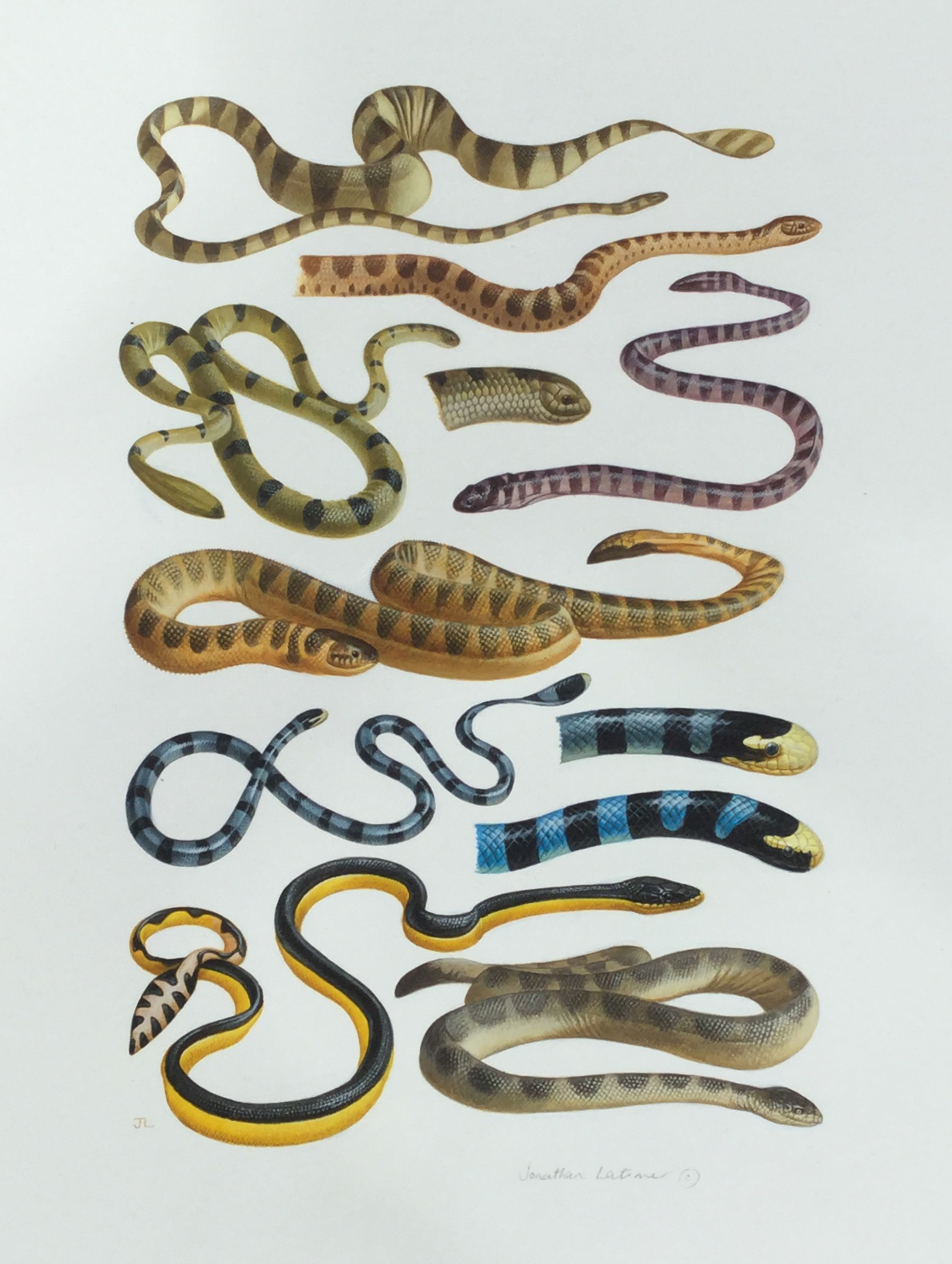This image showcases a vibrant and detailed poster of various illustrated snakes against a gray background, each snake featuring unique colors and patterns. At the top, a full beige and brown snake with dark brown stripes stretches across the poster, while beneath it lies a beige snake with dark stripes. To the center-left, a full green snake with black stripes is depicted, sharing space with a purple snake featuring darker bands. In the middle, a blue snake with black stripes is flanked by two smaller blue and black snakes and a central gray snake head. Below this section, a striking green snake with black spots, a purple snake adorned with black spots, and a golden snake with dark green spots add to the diversity. Lower on the poster, there's a yellow and green snake with a polka-dotted tail, and right at the bottom,a predominantly white snake with gray stripes. The entire illustration is meticulously detailed, with a very small signature in the bottom right corner, showcasing the artist's craftsmanship.